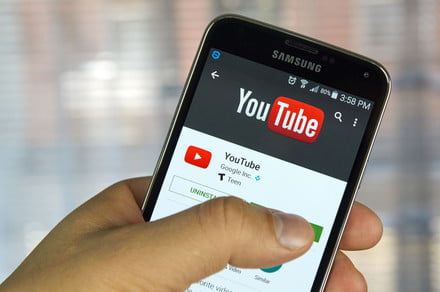A close-up image depicts a dark-skinned person holding a mobile phone in their left hand. The thumb is prominently placed on the screen, which displays the YouTube app page with the bold YouTube logo and the word "Google" also visible. The screen indicates an option to install or uninstall the app, with a green button partially obscured by the thumb, suggesting they are about to install it. The upper part of the screen includes black elements, with the rest being predominantly white, showing various installation options. The top status bar of the phone reads "3:58 p.m.", with the battery percentage also displayed, albeit blurred. The background of the image is an indistinct mosaic of light blue and pink hues, adding a subtle, abstract touch to the scene.